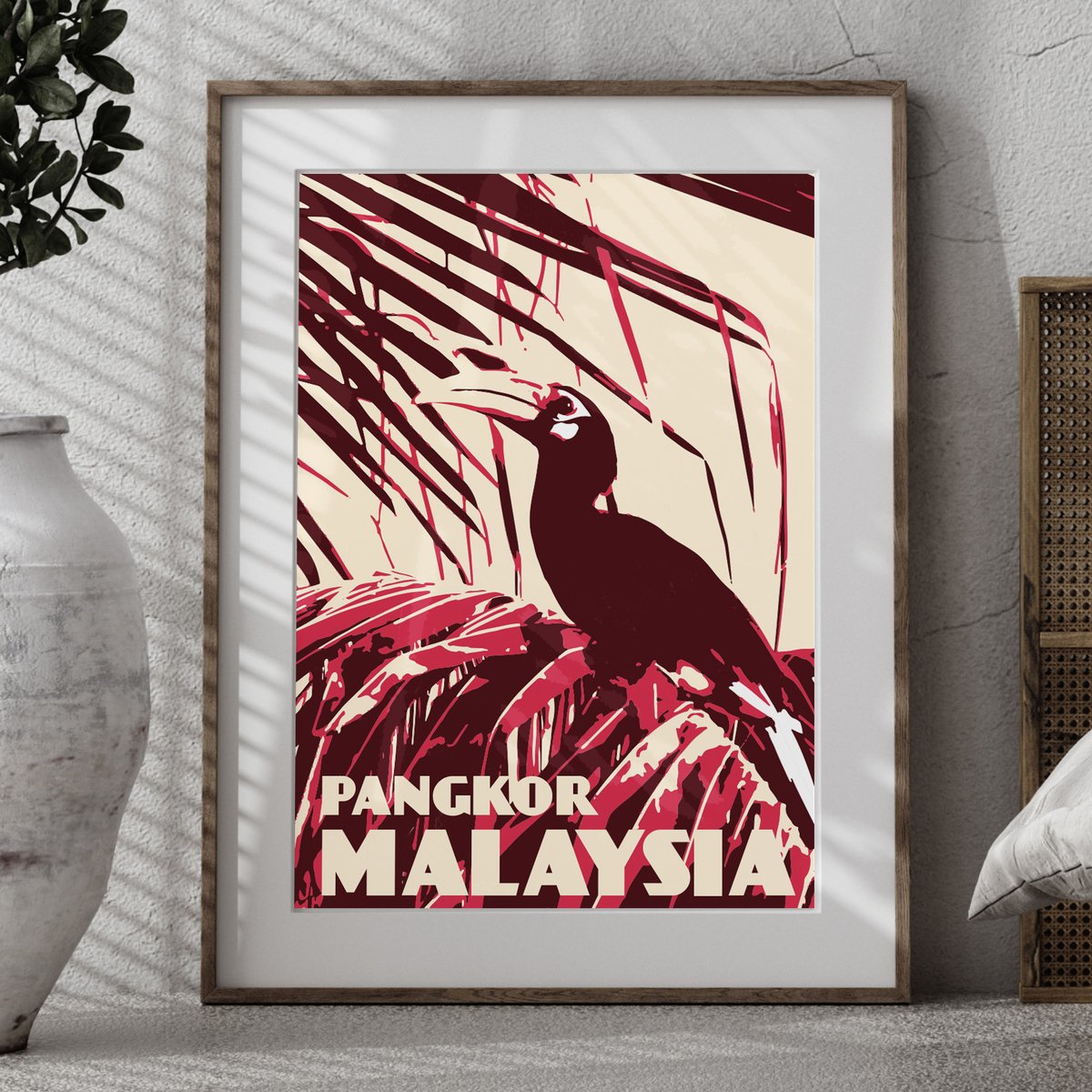This photograph captures a framed print leaning against a white wall in a home setting. The print features a detailed depiction of a black toucan with a long, slightly curved white beak and red accents on its beak, wings, and tail feather. The toucan is centered in the image, surrounded by green leaves with red highlights. At the bottom of the print, yellow text reads "Pangkor, Malaysia," hinting at the bird’s native environment. The artwork is enclosed in a brown frame with a white border. To the left of the print, a large potted plant slightly encroaches into the frame, while a vase also rests on the bottom left, and a small section of a throw pillow is visible on the bottom right. The lower portion of the image includes a carpeted floor, accentuating the cozy, indoor atmosphere. The color palette of the scene is primarily reds, blacks, whites, browns, and greens, creating a warm and inviting aesthetic.